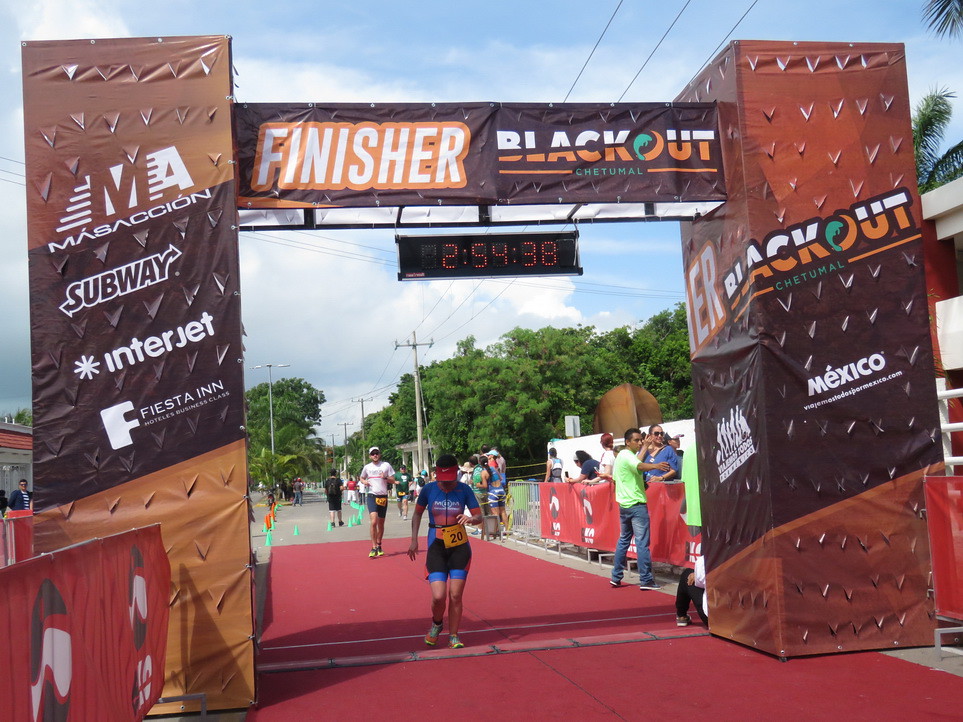The photograph captures a vivid and dynamic scene of a race finish line. Central to the image is a runner, contestant number 20, adorned in a blue and red outfit with black accents, and sporting a red Nike visor. The runner is crossing a red carpet that denotes the finish line, and above them, a timer reads "2:54:38". Flanking the finish line are two large pillars covered with logos of sponsors including Subway, Interjet, Fiesta Inn, and other brands. The top of the finish line structure prominently displays the words “Finisher Blackout Chetumal,” with additional text on the right side indicating sponsorship from Mexico. The background reveals a clear blue sky with a few white clouds, green foliage, and some electric lines, adding to the vibrant atmosphere. Other runners and supporters are seen in the distance, contributing to the bustling energy of the event.